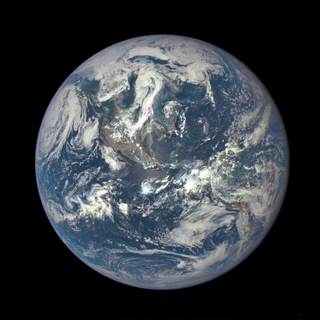This is a photograph of Earth taken from outer space, showcasing our planet against a completely black, featureless background. Dominated by the deep, dark blue of the oceans, the image also highlights swirling patterns of dense white clouds that resemble marble. Notably, the Earth’s land masses, including North America in the top left and South America in the bottom right, are partially obscured by these clouds. A distinct pocket of thick, swirling clouds can be seen in the top left. Some regions display darker shades of blue, while other sections are lighter. Small bits of brown and green land masses peek through the clouds, with a notable brown area in the center that appears to be a mountain, although most of the land is heavily blanketed by clouds. Overall, the image emphasizes the vastness of Earth's water, the intricate cloud formations, and the minimal visibility of the land beneath.